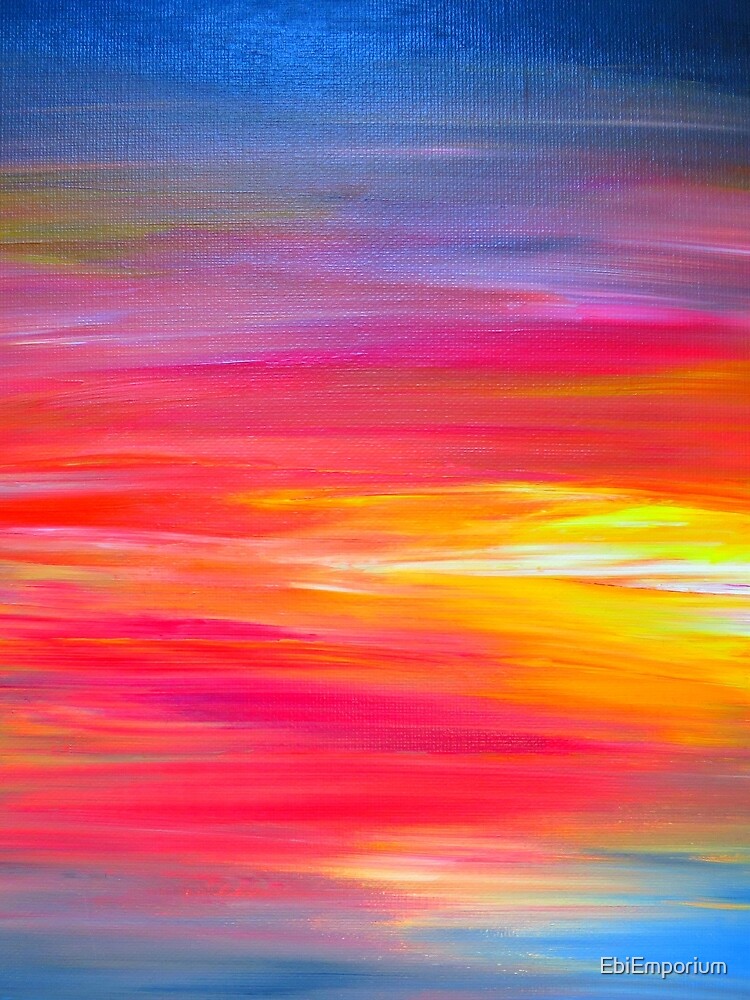This painting by EB Emporium on a canvas features a stunning array of colors arranged in horizontal layers, creating a vibrant and abstract masterpiece. Starting from the top, the image begins with a deep dark blue, transitioning through lighter blue hues, and then into dark and neon purples. Following these purples, the colors shift into a spectrum of oranges and reds, which blend into yellows interspersed with tints of white. The central part of the painting sees a repetition of purples, reds, and pinks, which fade again into the orangish yellows. As the layers descend further, the painting transitions back into shades of blue and purple, eventually concluding with a light blue at the very bottom. The bottom right of the canvas carries the artist's signature in white letters: "EB EMPORIUM." The entire piece captures a sense of a sunset in an abstract manner, with its rich collage of colors merging seamlessly together.